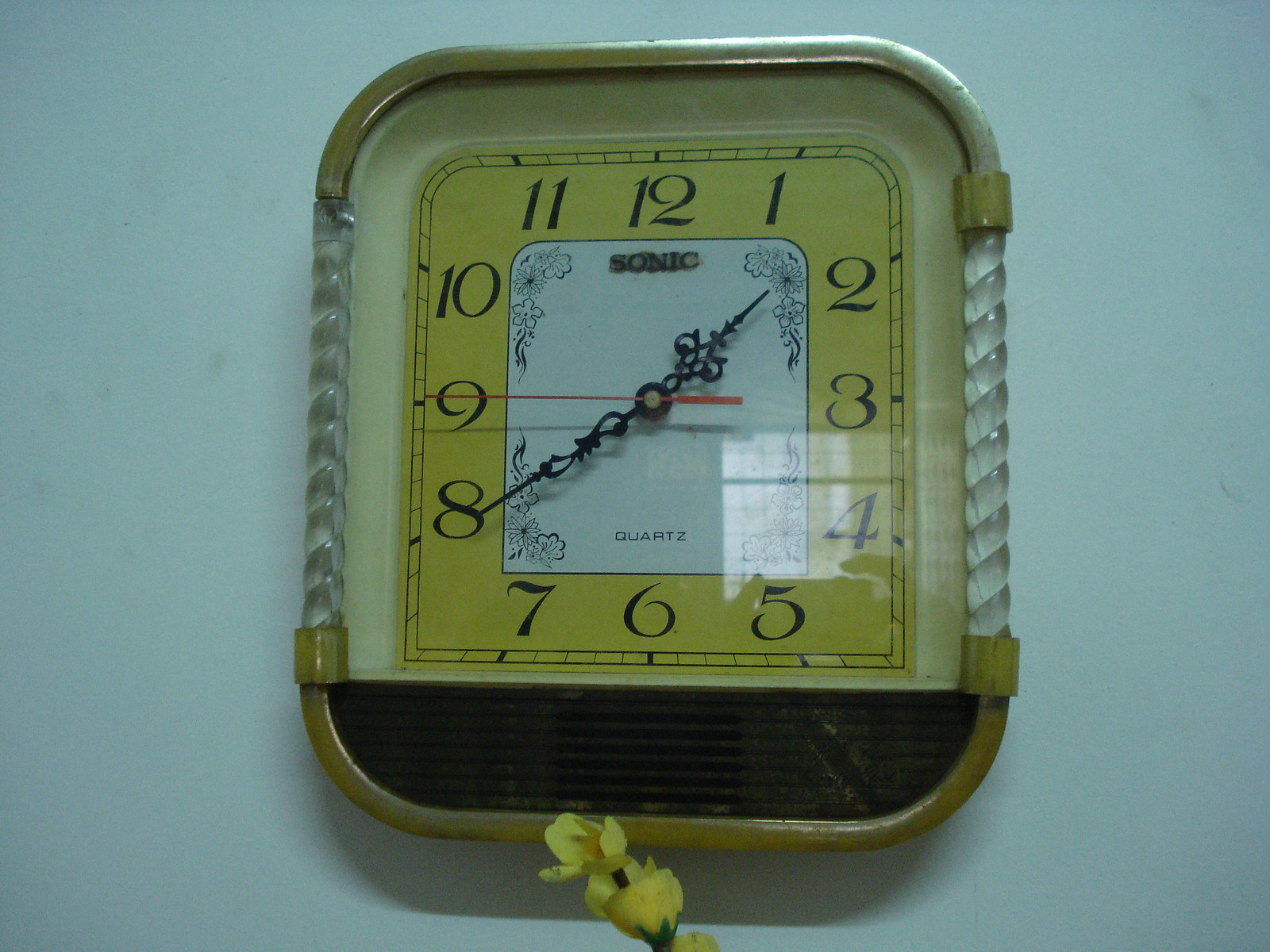Displayed in the color photograph is a vintage wall clock from the 70s or 80s, mounted on a white surface marred by light gray smudges. The clock has a rectangular shape with rounded edges and is encased in a gold metal border. This border features clear, braided plastic pillars on either side, giving it an intricate look. Covering the face is a reflective glass.

The clock face itself offers a striking combination of light and mustard yellow hues, with black, ornate numbers ranging from 1 to 12 clearly visible. Additionally, the words "SONIC" in bold all caps are positioned under the 12, and "QUARTZ" in smaller, non-bold all caps is shown just above the 6. The ornate black hands are supplemented by a red-tipped second hand, which stands out against the yellow background. A small portion of a yellow plant peeks into view from below the clock, adding an extra touch of color to the scene.